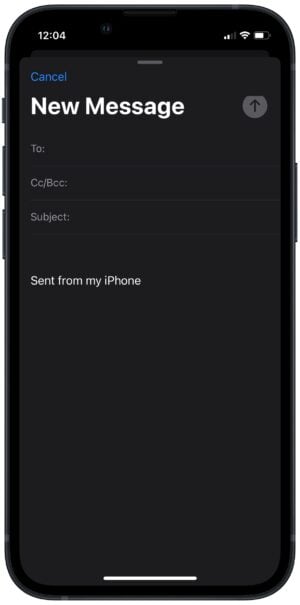The image appears to be a stylized representation of a mobile phone screen, not photorealistic but clear enough to identify key elements. The screen has a black background with curved edges. At the bottom center, a white horizontal line extends about a third of the way across. In the top left corner, white text reads "1204," while in the top right corner, icons indicate three bars for signal strength, three bars for Wi-Fi, and a nearly full battery.

Below these icons, a thin, narrow bar is centered and grey in color. On the left side of the screen, the word "Cancel" appears in blue. At the top center, "New Message" is written in white, accompanied by a grey circle on the right containing a black up arrow. The top part of this circle is slightly cut off.

Further down, three input fields labeled "To," "CC/BCC," and "Subject" appear in grey with thin grey lines separating them. Below these fields, the message body itself is displayed in white text stating, "Sent from my iPhone."

On the left edge of the phone, three buttons are visible: a small button at the top and two longer buttons beneath it. On the right edge, there is a longer rocker button. The bottom edge of the screen is faintly outlined against a lighter black background, though it is challenging to distinguish.